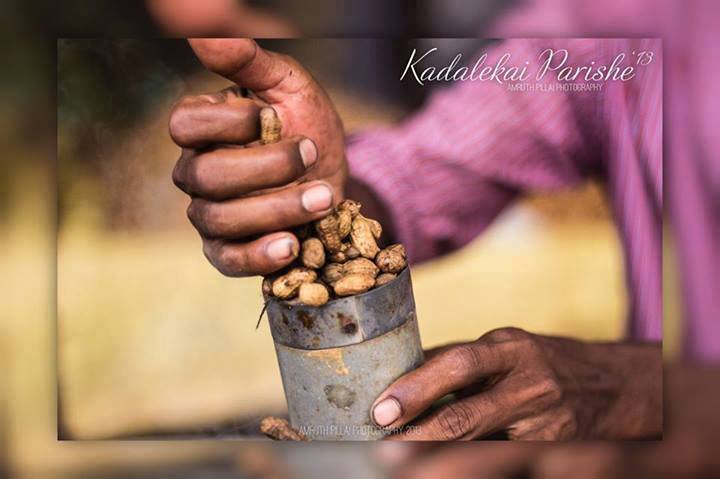The close-up, color photograph captures a person's hands actively placing peanuts into a tarnished, pocket-sized, metal canister, which appears old and well-used, suggesting it might be a favorite. The individual is wearing a long-sleeved, pink and white striped shirt, indicating a casual or everyday scene. The hands, worn and work-roughened, suggest a lifetime of manual labor or age. The canister prominently displays the inscription "KADLEKAI PARISHE" in flowing cursive, with additional but smaller text below it, including "A.M. FUTH PILLAI PHOTOGRAPHY." The background of the photograph is blurred, emphasizing the subject's hands and the canister, while an artistic effect frames the image with a larger, out-of-focus border.